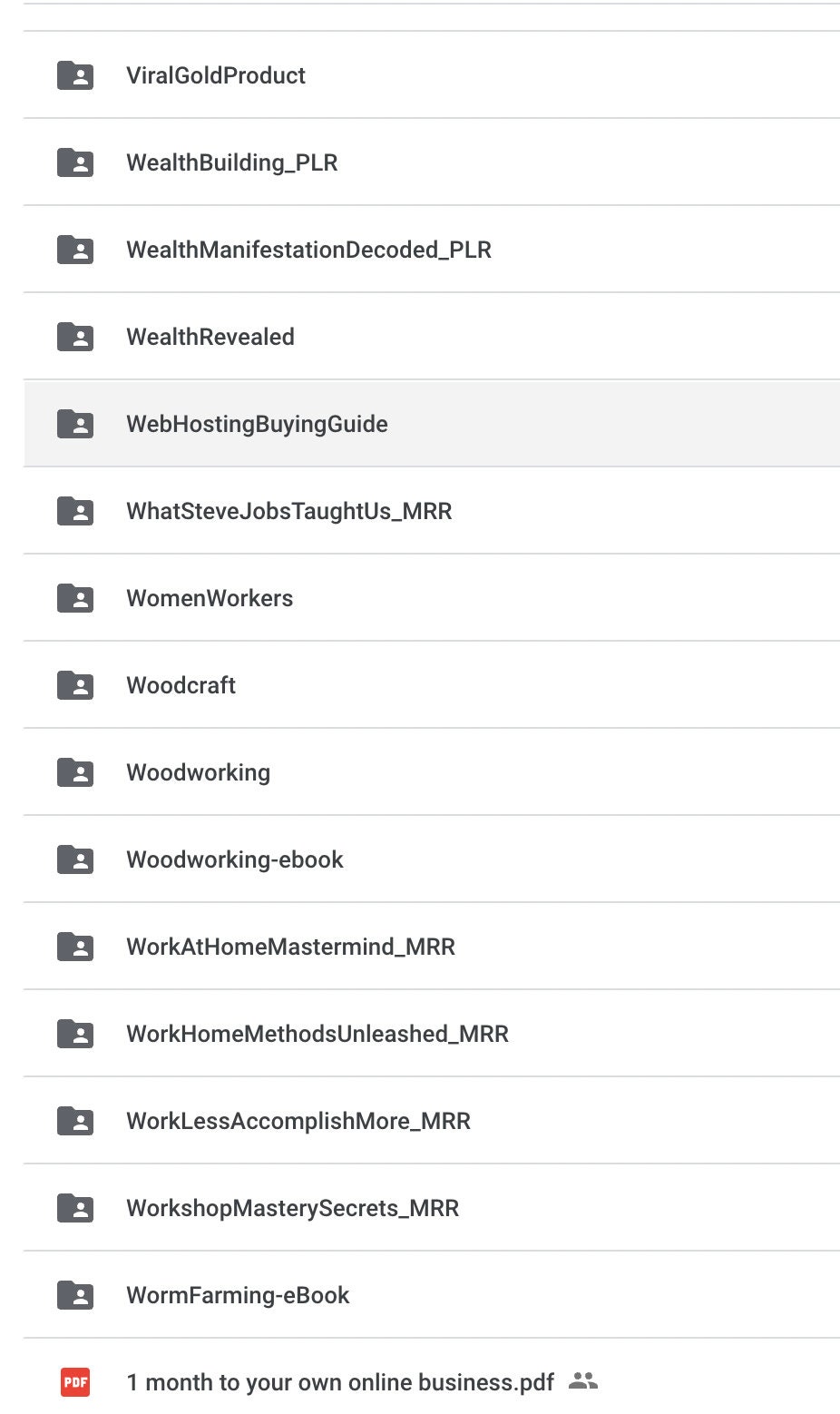The image displays a comprehensive page of menu options, each represented by a file icon featuring a person symbol. The listed options include:

1. Viral Gold Product
2. Wealth Building (Underscore PLR)
3. Wealth Manifestation Decoded (Underscore PLR)
4. Wealth Revealed
5. Web Hosting Buying Guide
6. What Steve Jobs Taught Us (MMR)
7. Women Workers Woodcraft
8. Woodworking (Dash eBook)
9. Work at Home Mastermind (Underscore MRR)
10. Work Home Methods Unleashed (Underscore MRR)
11. Work Less Accomplish More (Underscore MRR)
12. Workshop Mastery Secrets
13. Worm Farming (Dash eBook)

On the left-hand side, there is a small red square labeled "PDF" and a note that reads "One Month to Your Own Online Business.pdf." 

This might be a menu for files related to multi-level marketing or online business resources.